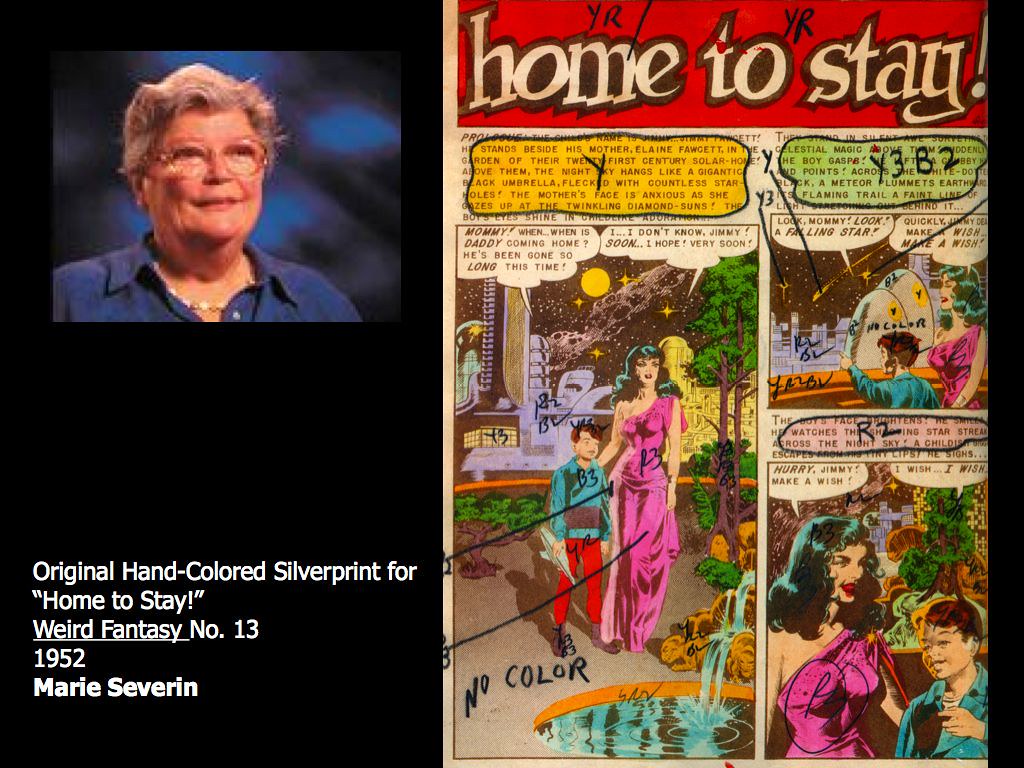The image is divided into two sections. On the left-hand side, set against a black studio background, there is a photograph of a smiling woman with short wavy gray hair, clear-framed glasses, and a blue button-up shirt with a collar. Below the photo, text reads: "Original hand-colored silver print for 'Home to Stay!' Weird Fantasy No. 13, 1952 Marie Severin." 

On the right-hand side, there is a close-up of a page from a comic strip. At the top of the comic page, inside a red box, it says "Home to Stay," but someone has drawn black markings over the text, adding "YR" over "home" and a "Y" between "to" and "stay." Below this, there are several comic panels, including a highlighted yellow box with a "Y" inside it. The comic depicts a woman and a boy, with labels "R3" and "B3" respectively, and dialogue bubbles where the boy calls the woman "mom" and is identified as Jimmy.